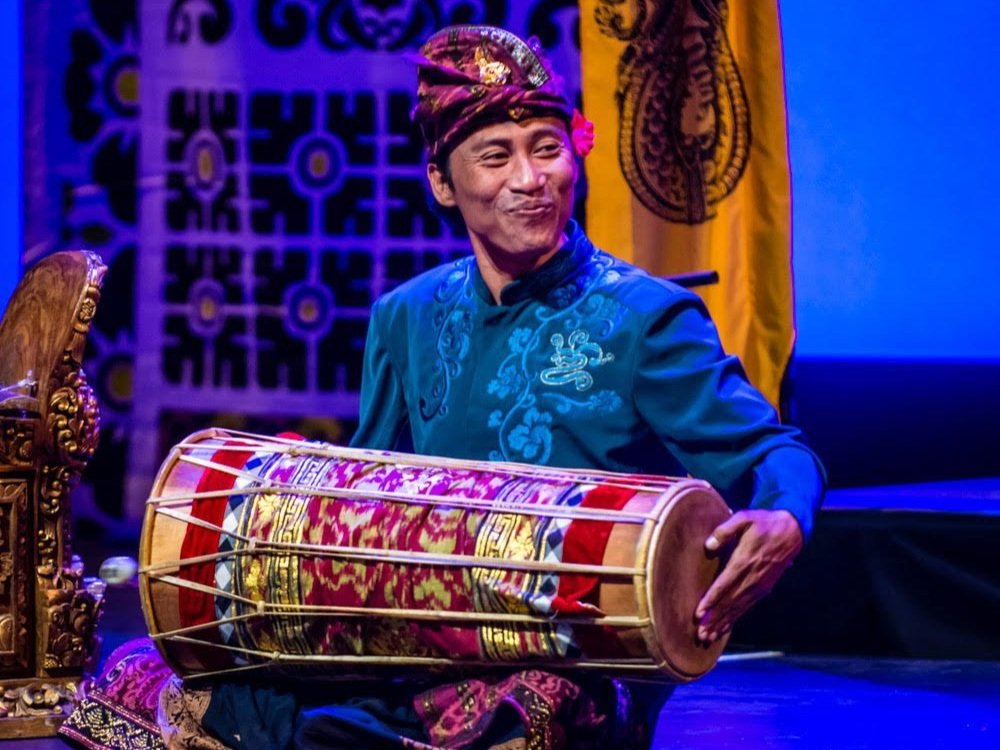In this vibrant landscape-oriented color photograph, the subject is a Japanese musician, Gamilan Gong Kebyar, captured mid-performance while seated in the center of the frame. He plays a distinctive, elongated hand drum that narrows toward the right side, resembling a cylindrical object that tapers down. The drum, positioned horizontally across his lap, is ornately decorated with a tapestry featuring tie-dyed hues of red, blue, gold, and purple.

Gamilan Gong Kebyar is adorned in a long-sleeved, decorative blue tunic shirt with light green embroidered scrollwork, complemented by ethnic print fabric shorts partially visible near the bottom of the image. His head is wrapped in a turban tied from a purple and gold scarf, and his pronounced cheekbones accentuate his warm smile, with crinkled eyes as he looks and smiles toward the right side of the image.

The background is rich with detailed decor: a gold banner hangs prominently on the right side, while a blue and gold ornate object and a brown wood carving embellish the bottom left. Behind him, a blue and black ethnic patterned backdrop serves as the stage setting. This photograph, stylistically rooted in representational realism, captures the joy and cultural richness of Gamilan Gong Kebyar’s musical performance.